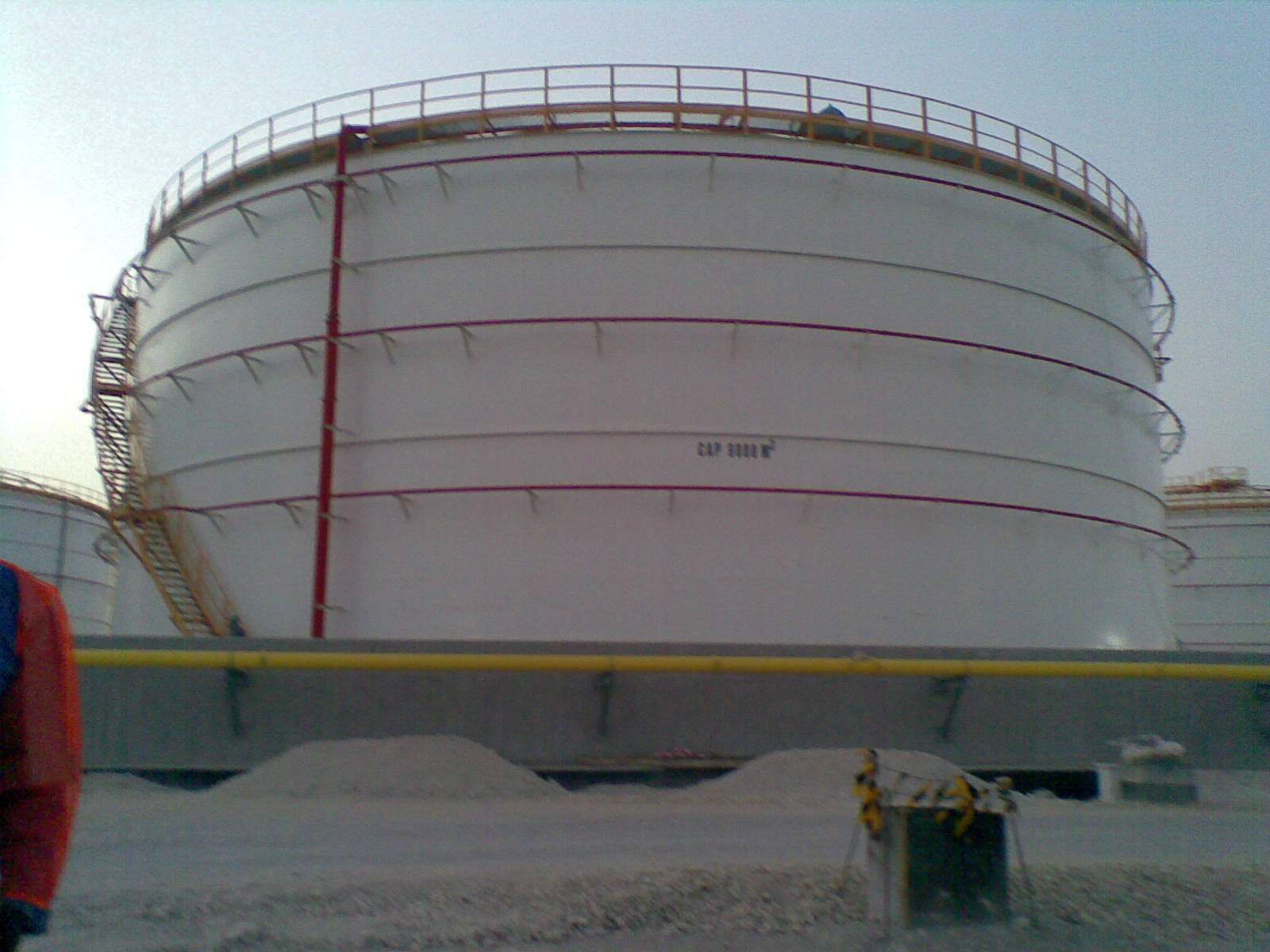The color photograph, albeit slightly out of focus and captured in landscape mode, depicts an industrial site, possibly near a port or shipyard. The centerpiece is an enormous round, white storage tank adorned with red safety rails around the top and silver handles on several attached red rims. The tank is several stories high and has a staircase on the left side ascending toward the top. Surrounding the base of the tank is a flat area covered with mounds of dark brown sand or similar material, possibly tailings.

In the foreground, there are metal brackets and a cinder block with yellow and black tape about two inches from the bottom right corner. A yellow handrail runs almost halfway up the photo, providing a median that separates different sections of the site. On the very left bottom corner, a person's left arm and shoulder, clad in either a safety orange or red jacket, are just visible, indicating another layer of industrial safety gear. 

Additionally, there seems to be some sort of yellow conduit running alongside the scene, supported by the visible metal brackets. The overall impression is of a large, operational storage site, with repeated structures and additional white buildings visible in the background, contributing to the industrial ambiance of the setting.